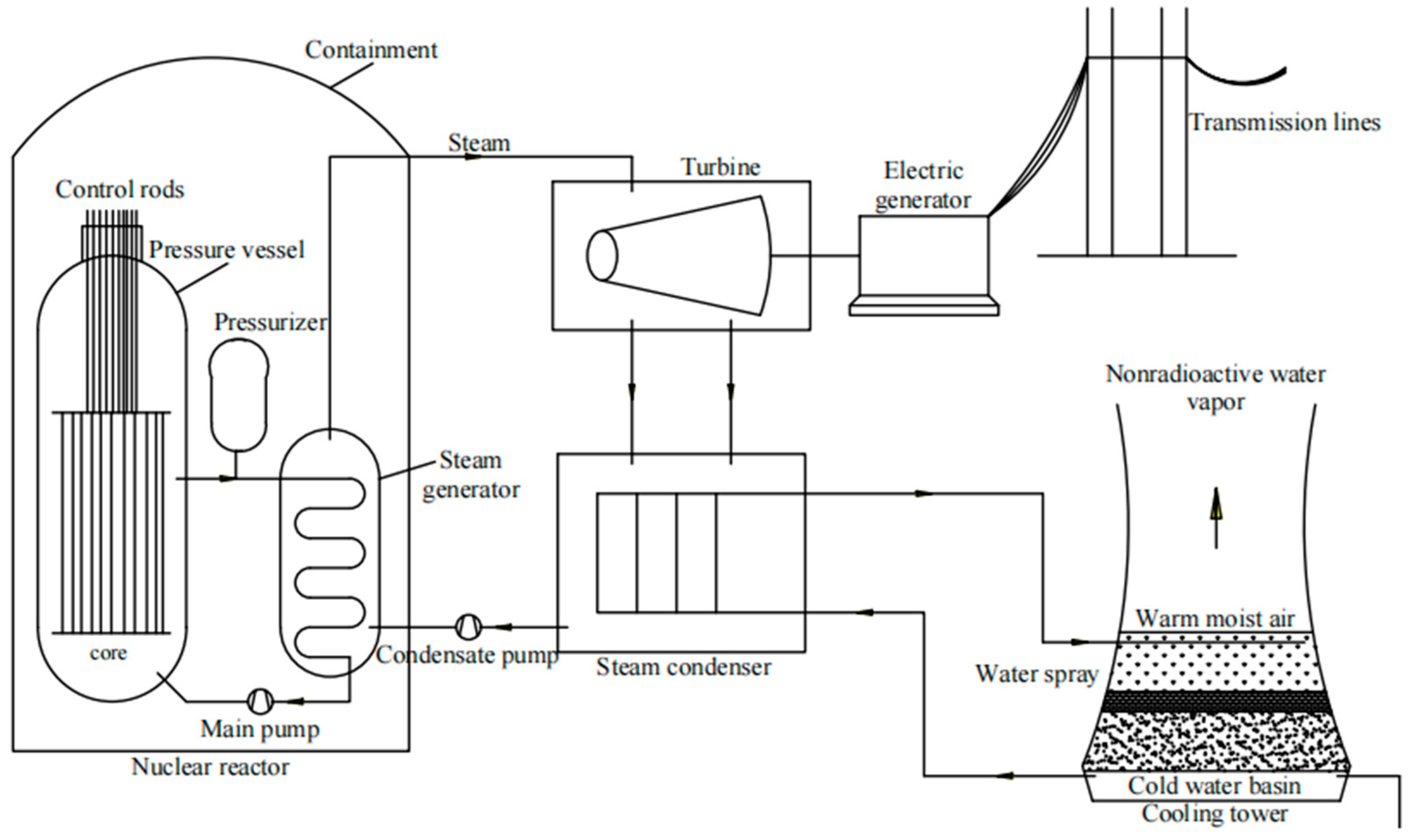This detailed educational blueprint illustrates the workings of a nuclear reactor. Beginning on the right, transmission lines connect to an electric generator, and a conical turbine. Steam from the turbine is directed to a pill-shaped steam generator. From there, the process continues to a pressurizer, a smaller oval shape, and then into a larger oval that houses the nuclear reactor's pressure vessel, core, and control rods within the containment structure. This is followed by a main pump that circulates the steam. The steam is then condensed in a rectangular steam condenser, after passing through a condensate pump. From the steam condenser, the diagram shows a progression to a cooling tower shaped like a beaker flask. The cooling tower includes a cold water basin at its base, and a water spray system above it. The system releases warm, moist air and non-radioactive water vapor, depicted with arrows pointing upward from a filtration system. This blueprint meticulously lays out each component, from the steam generation to the final cooling process, providing a comprehensive overview of a nuclear reactor's function.